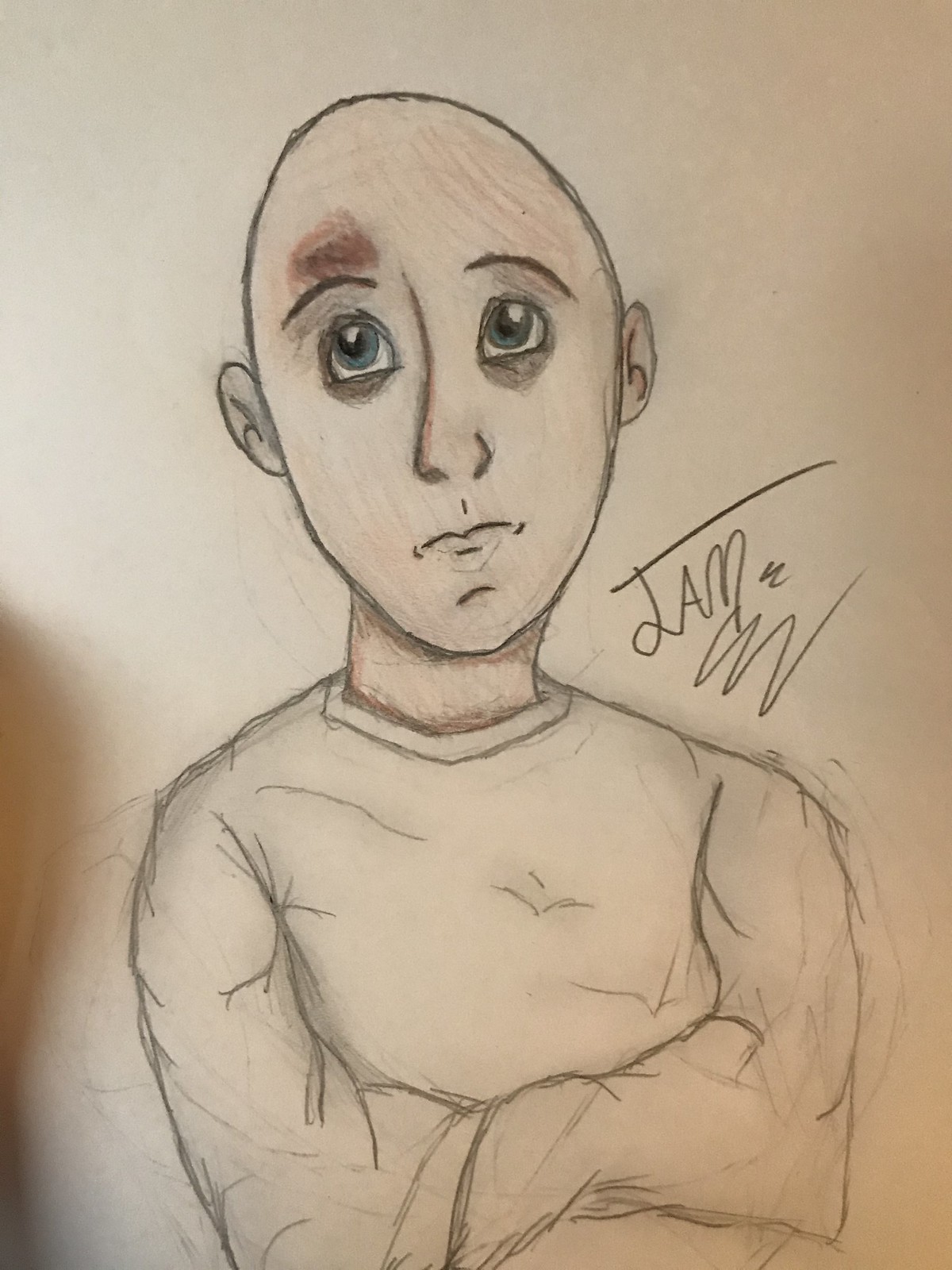The image is an indoor color photograph of a pencil sketch on a white sketchpad. The background is brownish-black, providing a dramatic contrast to the drawing. The sketch depicts a young, bald boy with blue eyes and an oval-shaped head. His eyes are slightly oversized and gaze upward and to the left, while his thin eyebrows curve downward, giving a concerned expression. Notably, there's a brownish patch or bruise above his left eye. His ears are simplistically drawn, and his mouth is a straight line, adding to his somber demeanor.

The boy's complexion is shaded with brown and tan colored pencils, providing depth and a lifelike quality. Darker shading under his eyes and around the wrinkles enhances the melancholic impression. He is adorned in a white, long-sleeved shirt that resembles a hospital gown or possibly a straitjacket since his arms are crossed tightly and no hands or fingers are visible.

To the right of the boy, there is a signature which appears to be "TAM" or "JAM," accompanied by squiggly lines beneath it. The sketch appears to be hand-held, indicated by a shadow cast on the left side. Overall, the detailed artwork emphasizes the boy's troubled expression and mysterious aura.